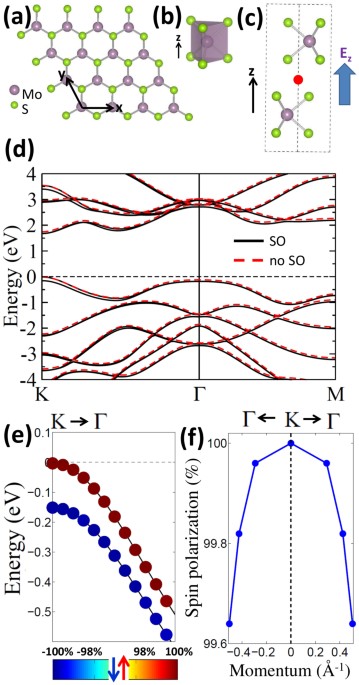This image displays a complex array of six labeled diagrams (A to F), each representing different types of data and scientific visualizations.

- **Diagram A:** Features a molecular structure with purple and green molecules interconnected to form a hexagonal pattern.
- **Diagram B:** Depicts a 3D triangular shape with green spheres at the vertices and a purple structure connected by edges.
- **Diagram C:** Shows a purple central dot with four extending lines, each terminating in a green sphere, depicting a simple molecular configuration.
- **Diagram D:** An energy graph with numbers ranging from -4 to +4 on the y-axis, possibly labeled with the Greek letter Sigma (Σ), K, and M. It includes red perforated lines illustrating energy variations.
- **Diagram E:** Another energy-related chart with a y-axis ranging from -0.5 to 0.1. It features blue and red dots aligned along gradients, with arrows indicating different directions.
- **Diagram F:** Presents a graph related to spin polarization and momentum, with a vertical scale from 99.6 to 100 and a horizontal scale from -0.4 to +0.4. The graph contains blue data points arranged along a plotted line.

The image encompasses various data representations, including line graphs, dot graphs, and 3D molecular models, all marked with relevant scientific notations and color codings such as red, blue, green, and purple. The visual information spans topics like energy distribution, molecular structures, and spin polarization.